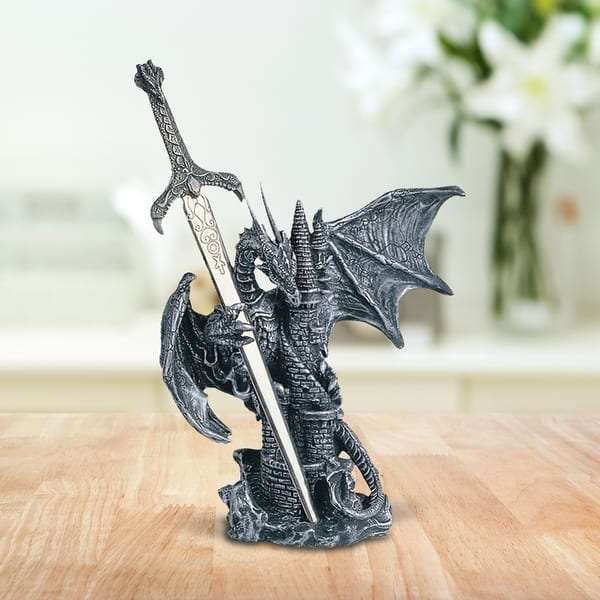The image showcases a detailed sculpture positioned on a light tan, wooden floor with visible intricate grain lines. The sculpture is crafted from a gray, black, and white material, possibly metal, clay, or polymer. It features a medieval-style dragon with its wings spread wide, holding a large sword in one hand and an ornate, tapering tower in the other. The sword, adorned with intricate designs and a dragon head at the hilt, extends taller than the dragon itself. The tower, resembling a stone pine cone at the top, wraps with a winding stairway and is about two-thirds the height of the sword. The dragon's tail coils around the base of the tower. Behind the sculpture, the blurred background reveals a vase of white flowers with yellow centers and a stack of books or other indeterminate objects. The dragon sculpture, a blend of fantasy and intricate craftsmanship, stands prominently in the foreground, emphasizing its elaborate details against the softly focused background elements.